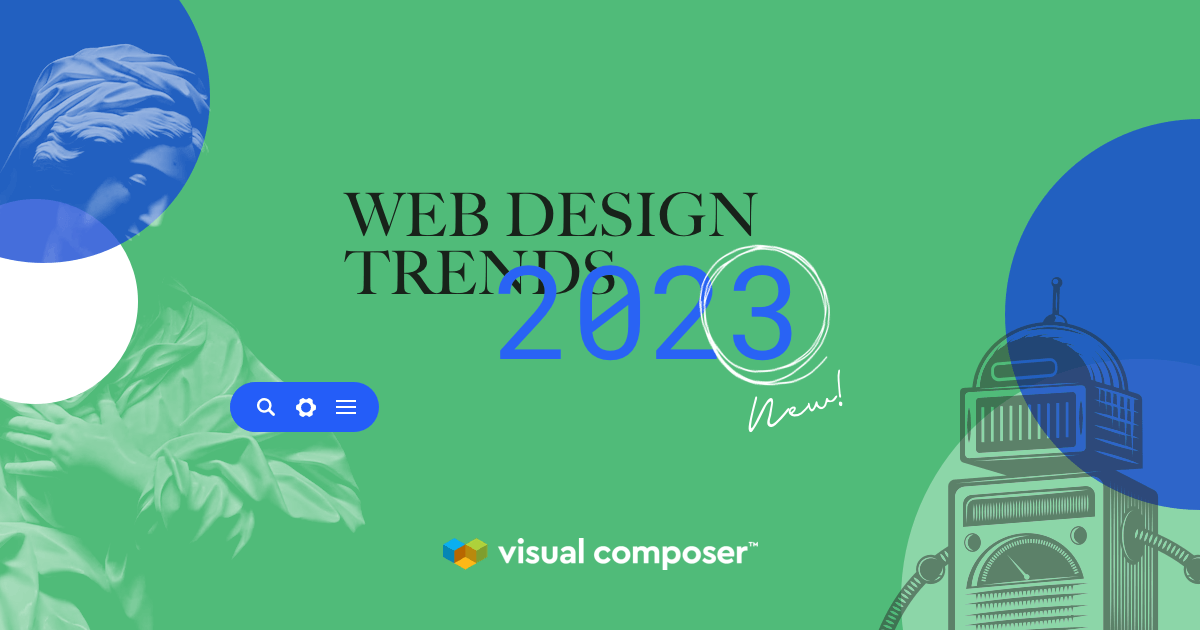This advertisement poster features a light green background and prominently showcases the text "Web Design Trends 2023" in the center. The phrase "Web Design Trends" is in black, while "2023" is displayed in large blue letters, with the number "3" circled in white and the word "new" written below it in cursive. The bottom middle of the poster displays the Visual Composer™ logo, accompanied by blue and yellow cubes.

On the left side of the poster, there are a series of circles: a blue circle at the top left and a white circle beneath it. Overlapping these circles is a faint image of a stone statue of a woman, gazing downward and to the right, with her left hand over her chest. Additionally, a blue pill-shaped icon containing three symbols—a magnifying glass, a cogwheel, and three horizontal lines—overlays her arm.

On the right side, a large blue semicircle is partially cut off by the edge of the frame, with a lighter green circle layered over it in the bottom right. Positioned over these shapes is a black-and-white outline of a robot featuring a rectangular body, a boxy head with a rounded top, and an antenna. This robot is situated near the bottom right corner of the poster.